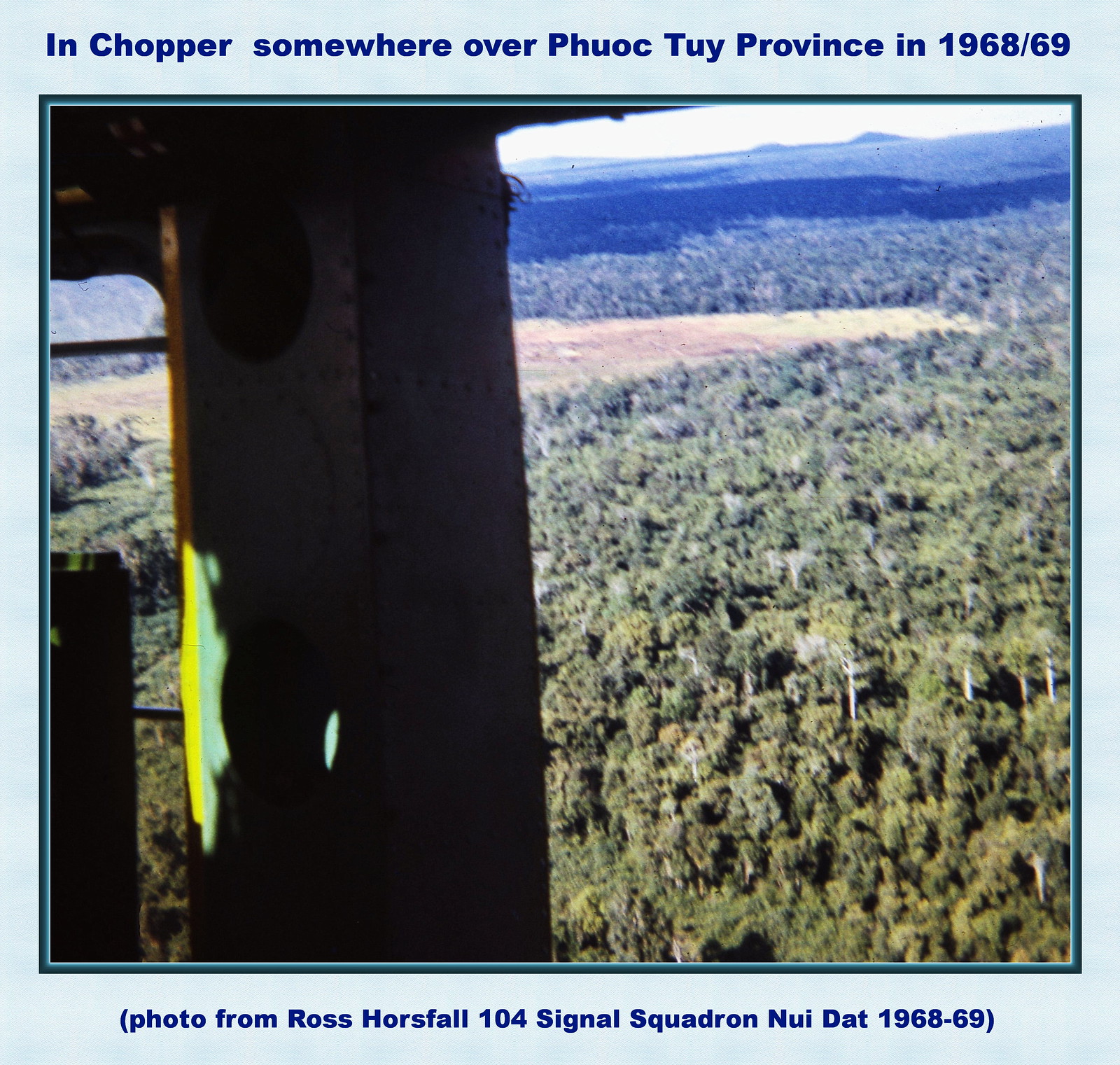This image resembles a square postcard, featuring a light blue border that surrounds a central photograph. At the top of the border, in blue letters, it reads "In chopper somewhere over Phuoc Tuy province in 1968/69," with "Phuoc Tuy" spelled p-h-u-o-c-t-u-y. Below the photograph, in parentheses, it states, "Photo from Ross Horsefall 104 Signal Squadron Nui Dat 1968-69." The photograph itself captures an aerial view from inside a helicopter, evident from the metal structure visible on the left side and doorway. The open view reveals a landscape of green trees interspersed with patches of tan-colored fields. In the distance, the terrain transitions into more fields and small mountains on the horizon, framed by the helicopter window on the right. The scene is bathed in natural light, emphasizing the contrast between the green foliage and the brown soil.